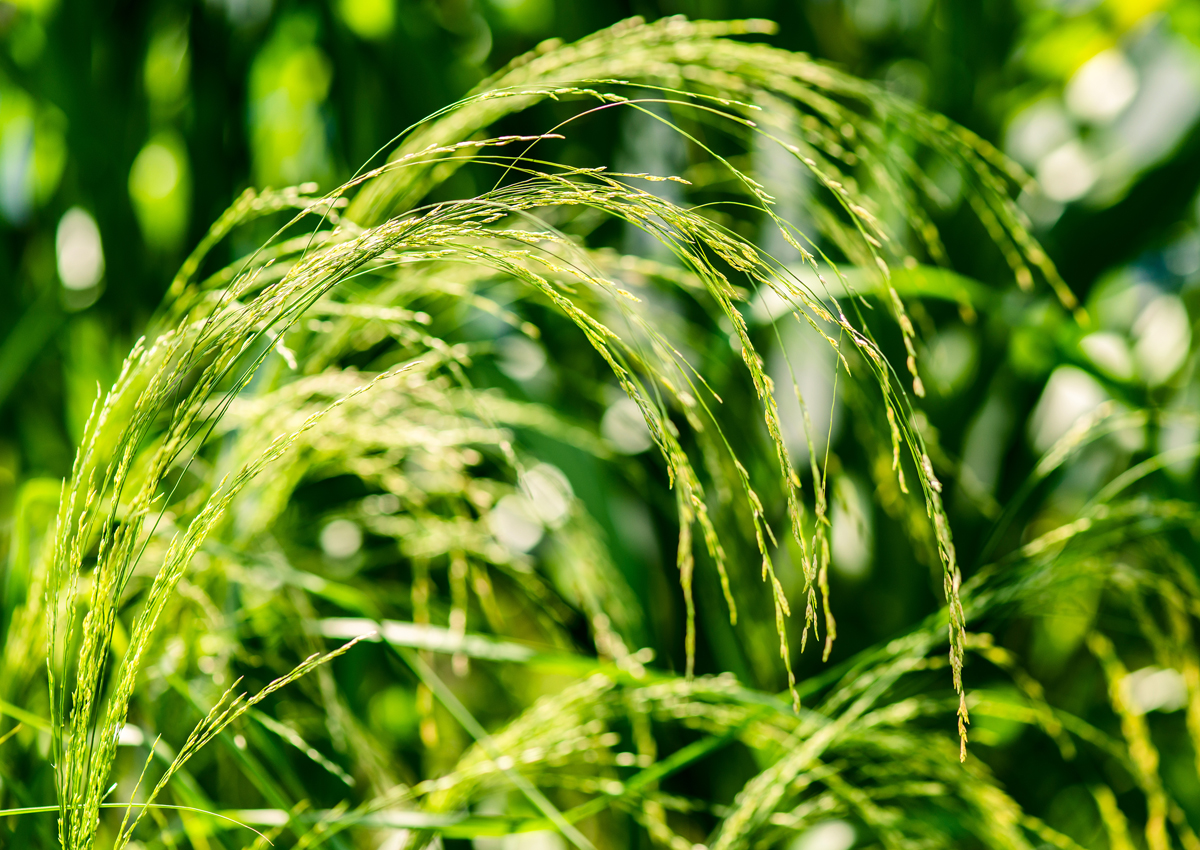This image captures a close-up of a plant taken outdoors during the day, set against a backdrop of blurred green vegetation with hints of white and yellow light filtering through. The photograph measures approximately 6 inches wide by 4 inches high and features the main subject—a delicate, wispy grass that emerges from the lower left-hand corner, extending upward and curving to the center-right. The plant consists of very thin, narrow stalks, some barren and dark green, while others are adorned with small seed pods, giving them a yellowish-green hue. The foreground plant is the image's focal point, exhibiting long, stringy strands that resemble grains of grass or a weedy plant like milkweed or ragweed. The background remains a soft green blur, accentuating the intricate details of the wispy grass highlighted by the bright daylight.